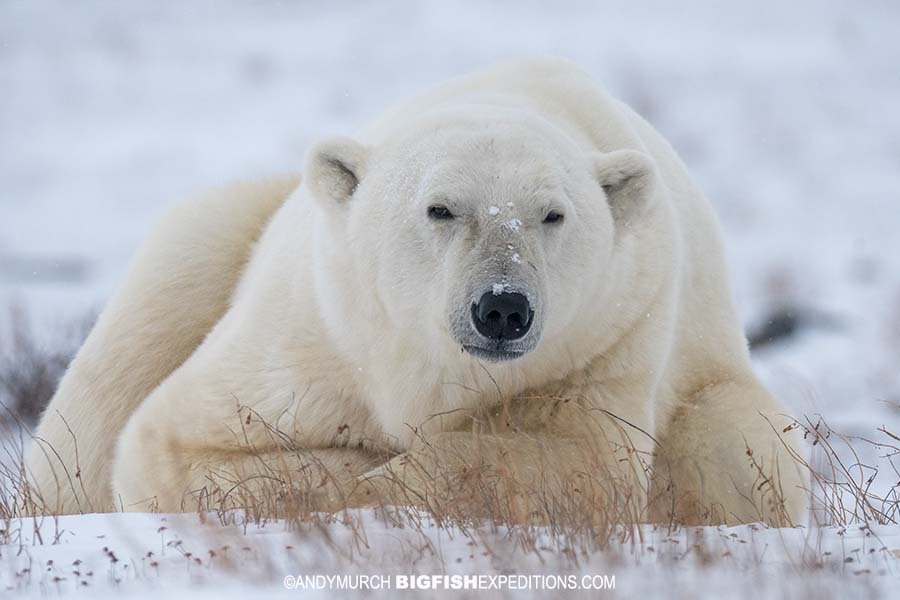This photograph captures a serene polar bear resting atop a snowy landscape. The bear, with its off-white fur and black nose and eyes, is lying down with its forearms stretched out in front, and its hind legs behind, gazing directly at the viewer with a calm, sleepy expression. Snowflakes delicately dust its nose and face, adding to its relaxed demeanor. The background is blurred and white, emphasizing the bear's in-focus presence, which dominates most of the frame. Sparse brown vegetation, just peeking through the snow, is visible in the foreground. At the bottom of the image, a copyright notice reads “Andy Murch, bigfishexpeditions.com,” indicating the photographer and his website. The overall scene evokes a sense of tranquility and natural beauty.